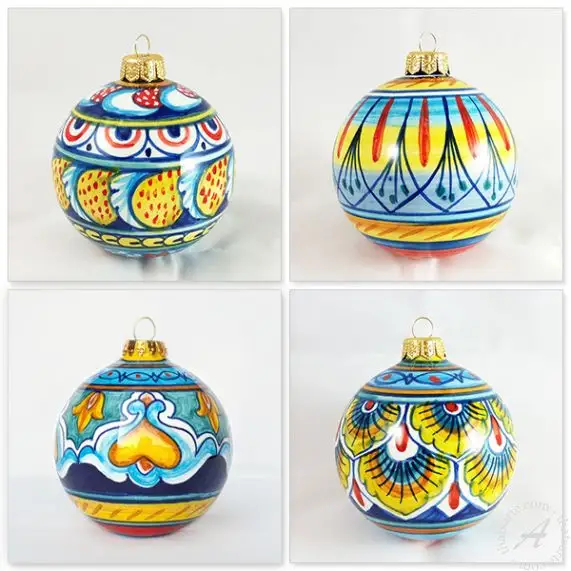In the image, four uniquely decorated Christmas ornament balls are arranged in a square grid, each occupying its own quadrant. The ornaments share a vivid color palette featuring dark blue, light blue, white, red, and yellow tones, but each boasts distinct designs.

The top left ornament showcases yellow circular bulbs with small red dots in the center, forming an intricate pattern. The top right ornament features thin elliptical lines, reminiscent of hanging lights, with blue bulbs accentuating the design.

In the bottom left quadrant, an orange heart takes center stage against a backdrop resembling blue water or clouds, exuding an abstract charm. The bottom right ornament, designed with a floral motif, has a blue center highlighted by an orange ring and a yellow outer edge, with a small, red central dot. Surrounding the central flower is a consistent floral pattern extending to the ornament’s edge.

All the ornaments are adorned with a gold hook and peg at the top, ready to be hung on a Christmas tree. Set against a pristine white background, the arrangement captures the festive essence and cultural richness of traditional Christmas decor, with each ornament reflecting delicate, possibly Mexican-inspired designs.